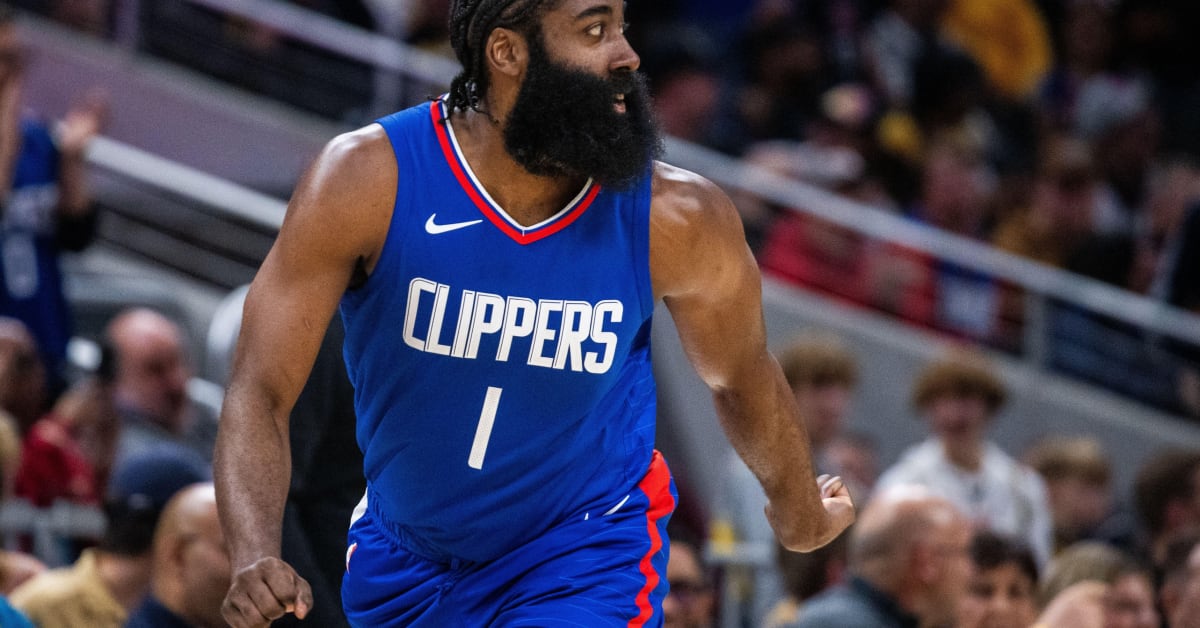The image depicts a professional basketball game featuring a player from the Los Angeles Clippers. The player, a black man with a notably bushy beard and mustache that connects into sideburns, is intensely focused on the court. His hair is neatly styled into red cornrows that dangle into a ponytail. Clad in a royal blue Clippers uniform trimmed with red and white, he proudly sports the number one and a white Nike swoosh on the upper arm of his jersey. In the midst of a run, his muscular arms are poised with one forward and one back, both held in fists. The photograph captures him from a close perspective, highlighting his sweat and athletic build, indicating mid-game action. In the blurred background, a sea of spectators in the indoor arena can be seen, all engrossed in the unfolding game.